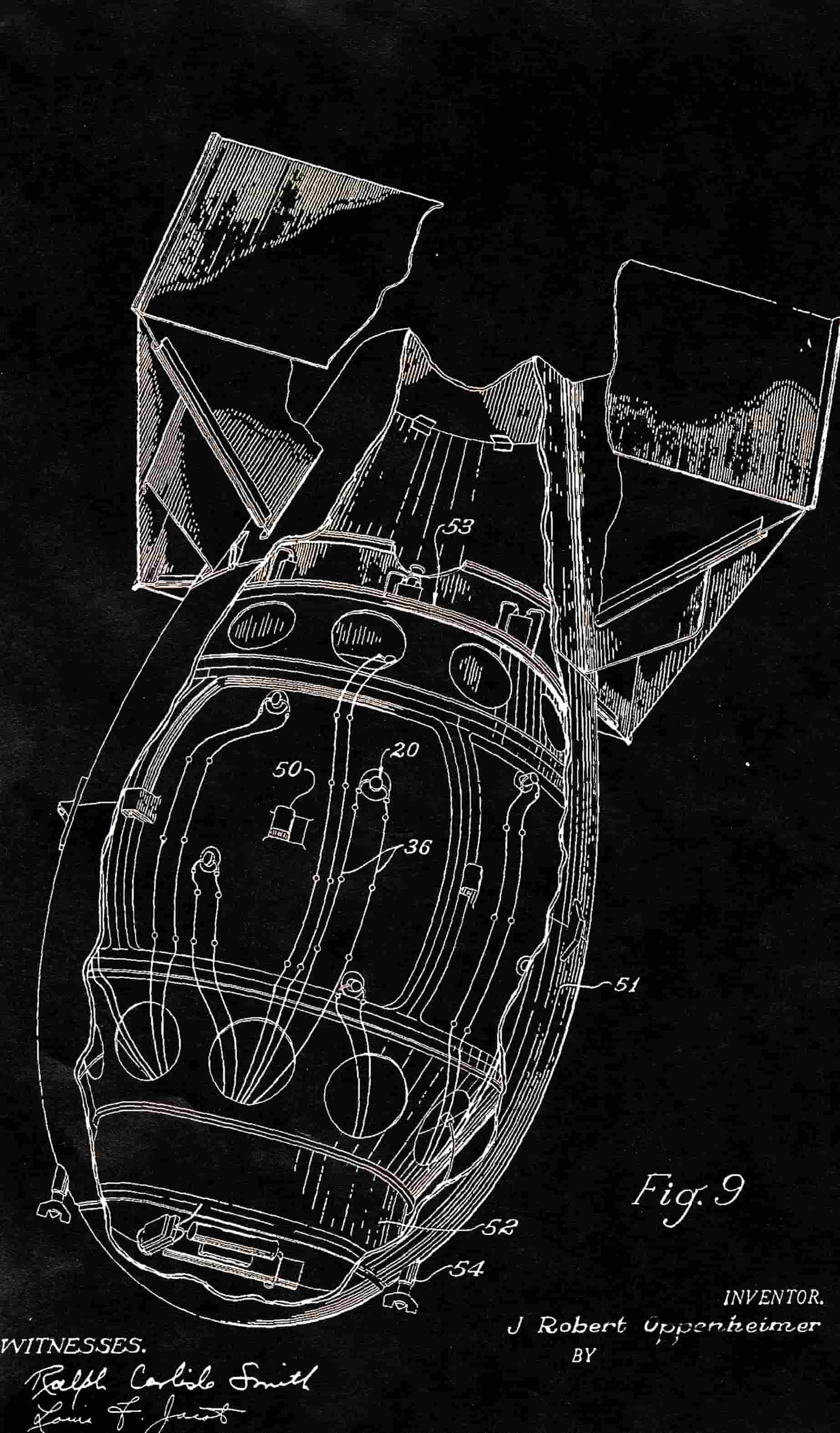The image is a detailed schematic of a large bomb, likely designed to be dropped from an airplane, presented as a white outline on a black background. The bomb has a thick, blimp-like central body with two fins forming a square shape at the tail. Multiple parts of the bomb are labeled with numbers, including 20, 36, and 50 through 54, though the corresponding key is not provided. The bomb is depicted nose down, emphasizing its aerodynamic design. In the lower right corner of the image, the text "Figure 9" is displayed, followed by "Inventor J. Robert Oppenheimer." Directly below this, there appears to be a partially obscured word that might read "Bye." On the lower left, there are two signatures for witnesses: one seems to be "Ralph Carlisle Smith," and the other is less clear, possibly "Louis Jarrett." The entire presentation suggests it could be an official or technical document, possibly a poster, highlighting the contributions of J. Robert Oppenheimer.